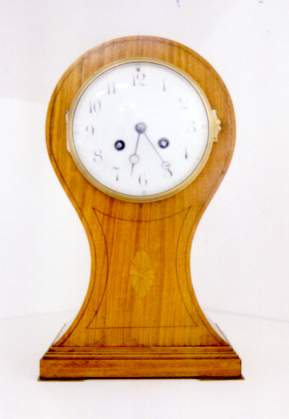This elegant mantle clock features a rectangular base crafted from lighter brown wood. From the base, the clock's structure curves gracefully inward at the center, then arches outward and upward, culminating in the display of the clock face. At the middle section of the clock, there is an oval-shaped decorative element resembling a leaf, intricately carved and adding a touch of sophistication.

The clock face itself is white and encircled by a gold band. This band is encased in glass, providing a protective yet stylish cover. The glass is hinged, allowing it to be opened via small gold brackets on either side. The clock’s numbers are in bold black, ensuring easy readability, while the minute and hour hands are also black for clear time telling. Additionally, there are two small black circles positioned just above the numbers seven and five, symmetrically placed on either side of the clock face.